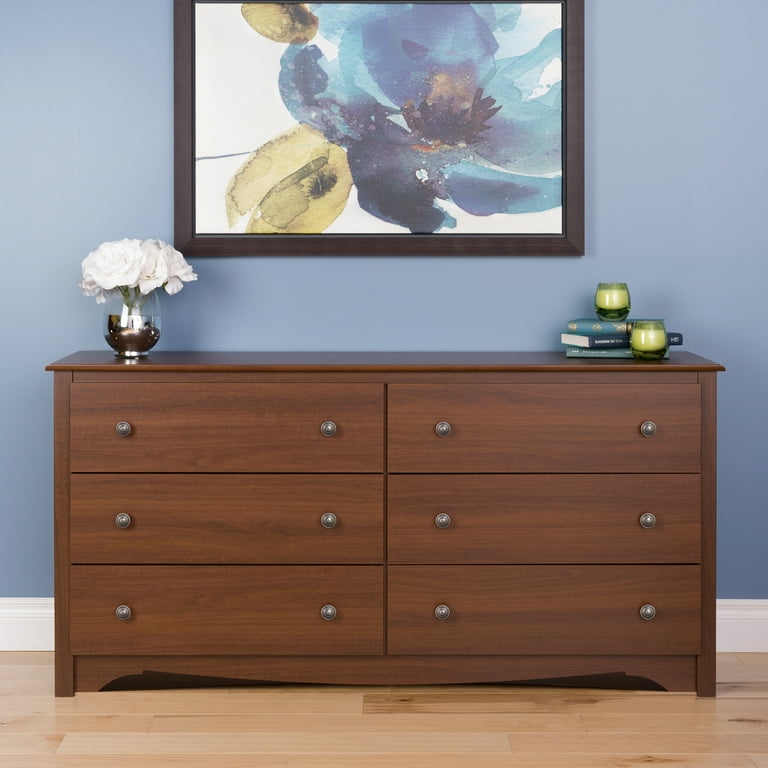This image depicts a wooden dresser, approximately four feet high, standing against a light blue painted wall with white floorboards. The dresser features six drawers arranged in two columns of three, each drawer fitted with two centrally placed silver metal handles. Positioned on a tan hardwood floor, the dresser is adorned with decorative items, including a glass vase filled with real white flowers on the left side, three books, and two candle holders on the right. Above the dresser hangs a dark brown wooden-framed painting, showcasing an abstract representation of flowers.